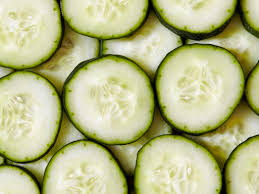This small, horizontally angled, color photograph is an extreme close-up of a series of cucumber slices laid out in a repeating pattern. The cucumbers are arranged in at least two layers, with the topmost layer displaying 12 full slices in a 3x4 grid. Surrounding these, the edges of the photograph reveal about 10 partial cucumber slices, either cut off by the frame or partially obscured by the overlapping layers beneath. Each cucumber slice features a dark green, almost black outer rim that transitions into a lighter, middle green layer, culminating in a very light, off-white center with a faint greenish tint. The seeds, barely visible, blend seamlessly into the pale centers, adding subtle detail to the crisp, fresh presentation. There are at least 20 cucumber slices visible, contributing to the visually appealing, grid-like arrangement.